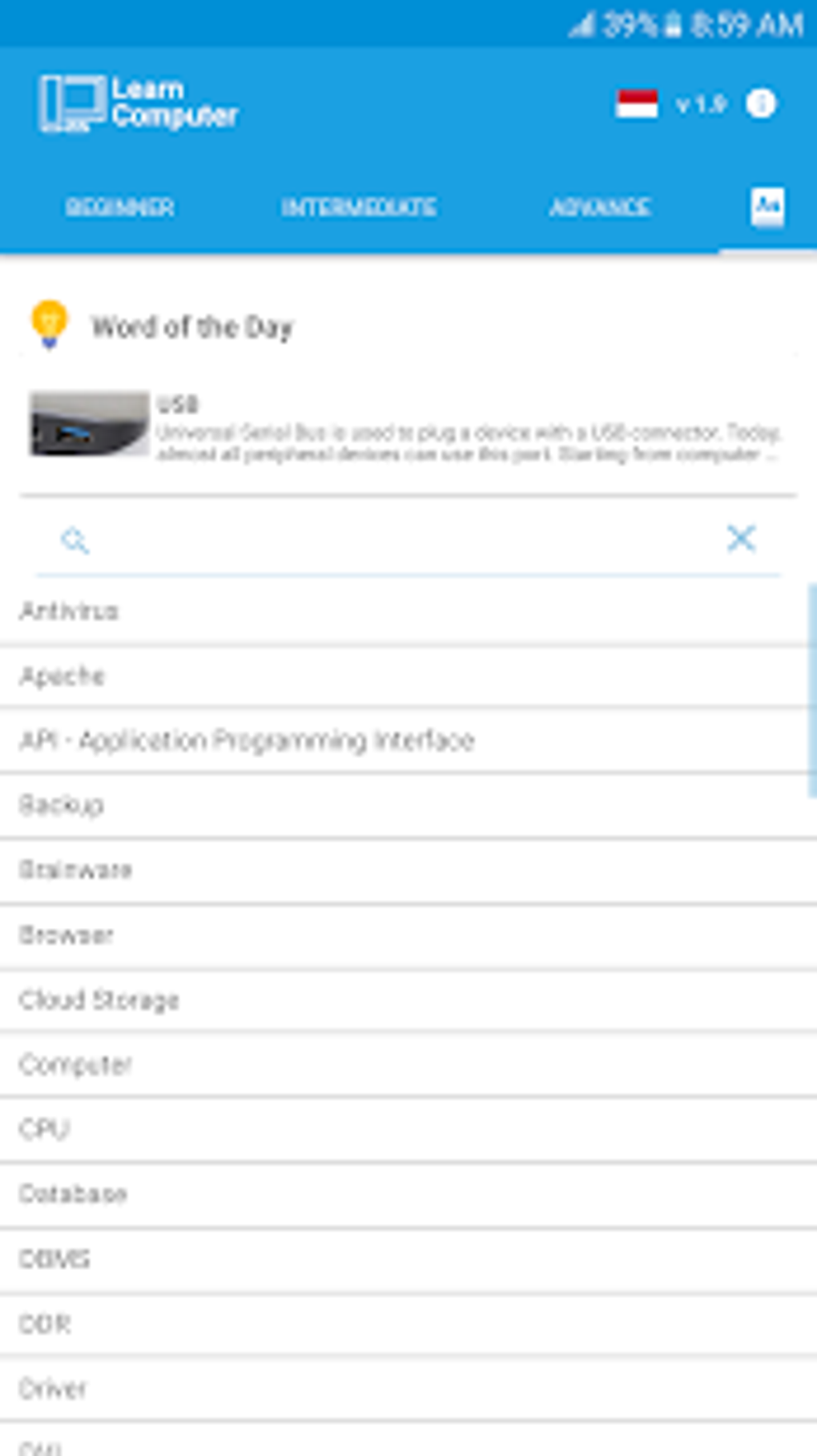**Descriptive Caption:**

The image is a screenshot taken in portrait mode, featuring a very blurry and difficult-to-read interface. The upper section of the image has a light blue background with a slightly darker blue stripe running horizontally from the upper left to the upper right. In the upper right corner, the display shows a 39% battery level and the time as something around 59 a.m.

In the second row, on the left side, there is text that seemingly reads "Learn Computer," and on the right side, there is a flag which appears to have red over white colors. Beneath this row, faint text seems to indicate some levels like "Beginner" and "Intermediate," though it's hard to decipher due to the light blue text on a light blue background. An icon is visible—possibly an award or a light bulb—next to the phrase "Word of the Day." The word of the day itself might be "USB," but the blurry text makes it hard to confirm.

Below this section, the background transitions to white, and there is a vertical white scrollbar on the right side, suggesting the content can be scrolled. The content here is organized in rows with headings that could likely be "Articles" and list terms such as "Apache," "API," "Browser," "Cloud Storage," "CPU," and "Driver," among others. The bottom left corner displays a word that is cut off, indicating more content is available by scrolling down.